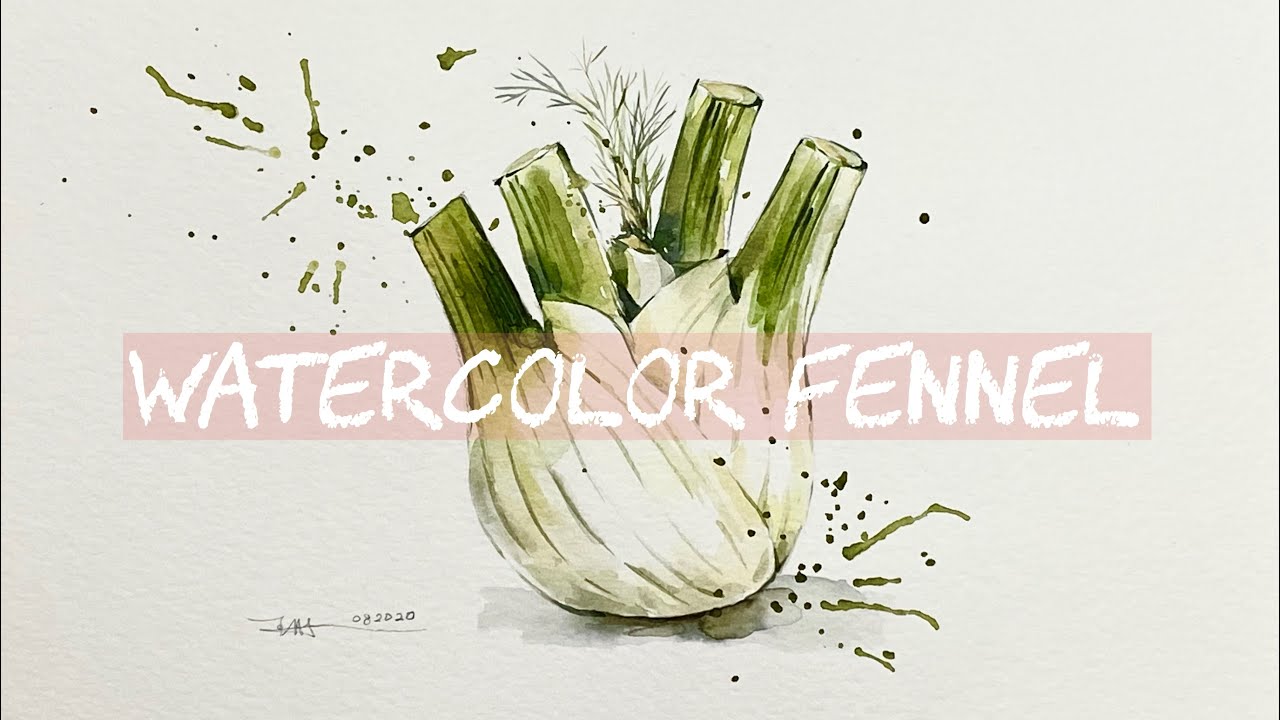The image titled "Watercolor Fennel" is a detailed painting that features a fennel bulb prominently at its center. The bulb is white and somewhat resembles garlic but with a distinct fennel foliage, including a small sprig of piney leaves emerging from its middle. There are four large green stalks, visibly cut off at the top as if they were trimmed by garden scissors, reinforcing its botanical identity. Around the bulb, small green specks are scattered, evoking the impression of an explosive burst of green liquid.

The central part of the image is overlaid with a pink banner, bearing the text "WATERCOLOR FENNEL" written in white, all-caps letters. This translucent banner spans most of the image's length and occupies about a tenth of its width. Additionally, there is an artist's signature accompanied by the date "08 2020," which appears in the bottom left corner, indicating that the painting was created in August 2020.

Overall, the artwork merges the anatomical structure of the fennel plant with an almost heart-like, organic explosion, creating a vivid and dynamic botanical illustration.